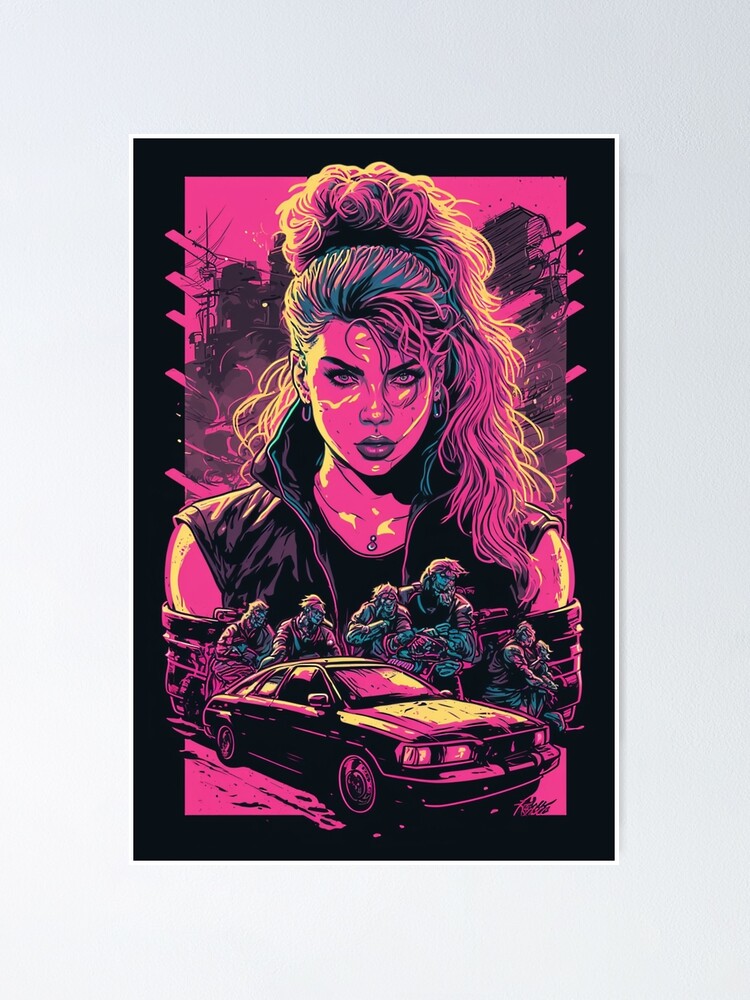The image showcases a striking pop art style poster set against a gray or off-white backdrop, possibly serving as a frame, with a thin white border followed by a prominent thick black border enclosing the artwork. The primary color dominating the image is a vibrant hot pink, complemented by accents of yellow and black. Central to the artwork is a girl taking up more than half of the space, gazing directly at the viewer with her piercing blue eyes. She has her hair styled in a cascading ponytail with wispy bangs and is adorned with paper clip-style hoop earrings and a pendant necklace. She wears a high-collared, sleeveless vest over a t-shirt, leaving her arms bare.

Her face, painted in hot pink with yellow highlights, pops against the background. Beneath or in front of her are cartoonish ape-like figures and a 1980s style four-door car, both rendered in the same bold color scheme of black with pink and yellow detailing. The entire composition involves a playful yet eye-catching juxtaposition of elements that epitomize the essence of pop art.